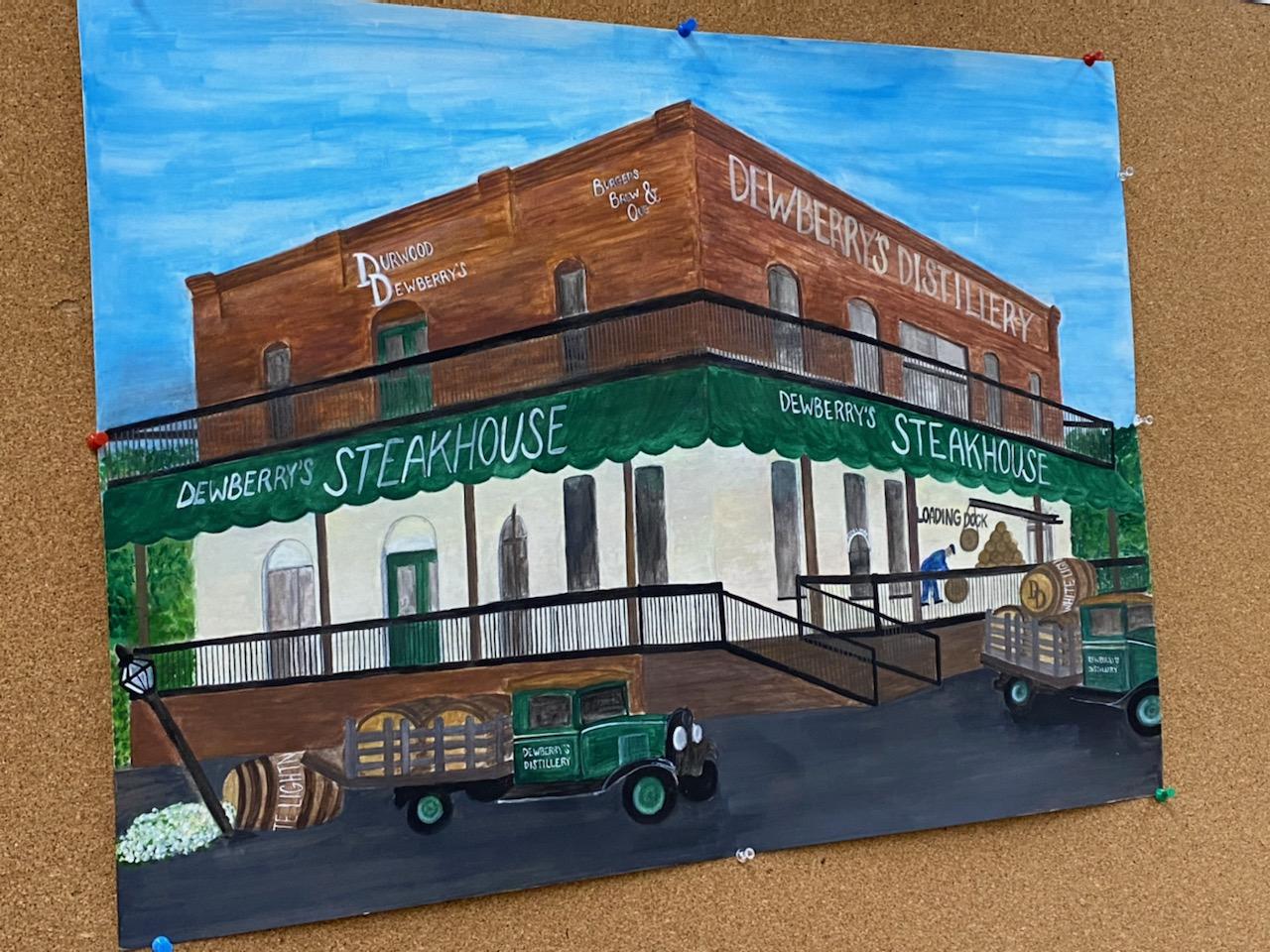The image is a detailed painting thumbtacked to a corkboard background, depicting a charming two-story building viewed from an angle, allowing both the front and side to be visible. The first floor of the building is painted white with a prominent green door and multiple windows, along with a green canvas overhang on either side that reads "Dewberry's Steakhouse." Above, the second floor features brown brick walls with windows and hand-painted signage that reads "Durwood Dewberries" on the left side and "Dewberries Distillery" on the right. In front of the building, set against a black road, two vintage green trucks with open trailers are present. One of these trailers has slatted sides and both trucks are loaded with large barrels, one of which has tumbled out, knocking over a black lamp post that now leans to the side. A small amount of white content spills from the fallen barrel, enhancing the quaint yet bustling atmosphere of the scene.